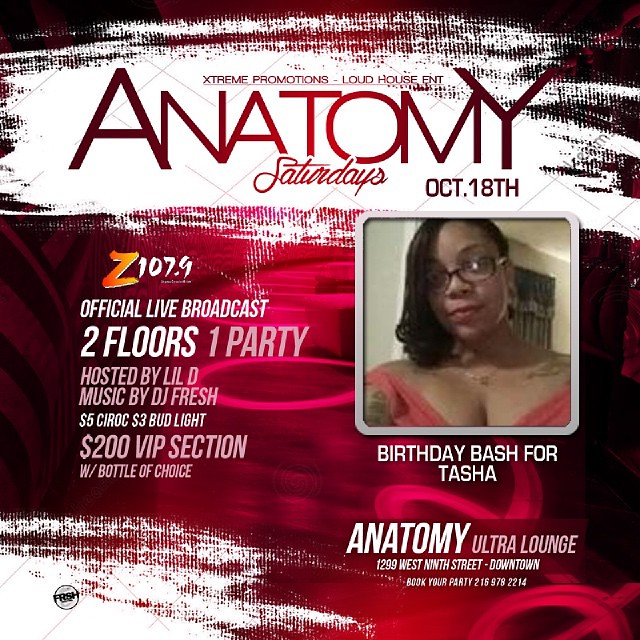This image is a detailed poster advertising an event at Anatomy Ultra Lounge, located at 1299 West 9th Street, downtown. The event is scheduled for Saturday, October 18th and is presented by Extreme Promotions and Loud House Entertainment.

Across the top of the poster against a white background, red letters read "Anatomy Saturdays." Directly beneath this, "October 18th" is inscribed in dark letters above a central photograph of a dark-skinned woman. She is wearing reddish-framed glasses and a thin, reddish dress that reveals some cleavage, accompanied by a gold necklace. Her hair is straight on one side and curls at the ends. 

To the left of the woman’s photo, the poster lists event details against a red background: "Z 107.9 Official Live Broadcast, 2 Floors, 1 Party, Hosted by Lil D, Music by DJ Fresh, $5 Ciroc, $3 Bud Lights, $200 VIP section with bottle of choice."

Under the woman’s photo, white letters announce, "Birthday Bash for Tasha." Additional information at the bottom provides a booking number: 216-978-2214.